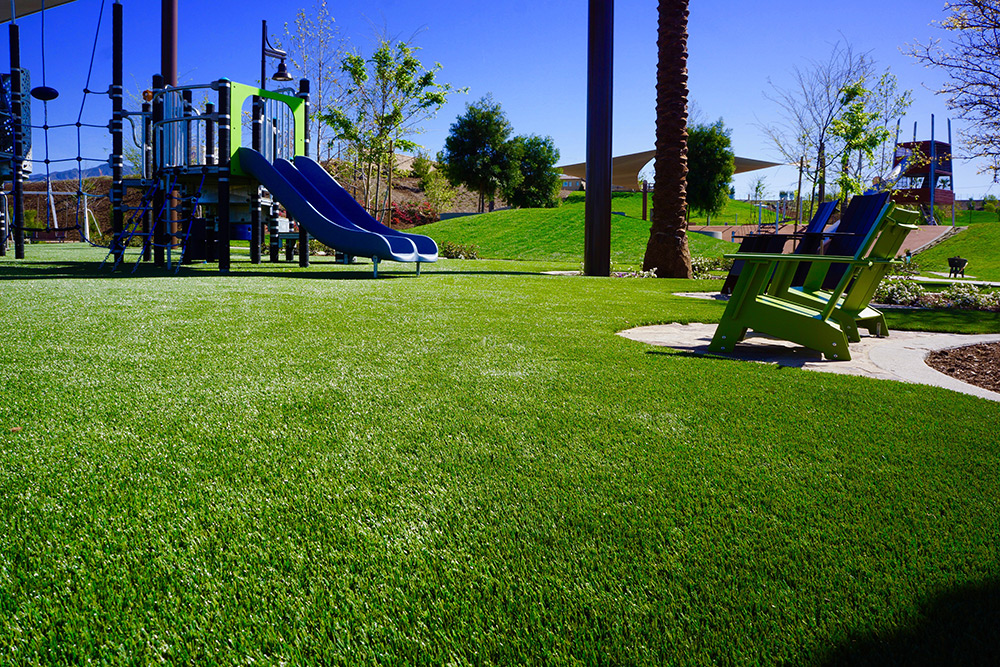The image captures a meticulously maintained playground, where the pure green grass is perfectly mowed, creating an immaculate ground cover that dominates the lower half of the picture. Located on the left side is an elaborate playset, primarily dark blue, with an inviting green archway leading to slides. The playset features not only blue slides but also rope structures for children to climb. To the right and slightly centered, a walking path weaves in and out, surrounded by a small flower planting area. Adjacent to the path are fancy lounge chairs in green and blue, seemingly designed for parents to watch over their children. The background of the photograph shows the trunks of several trees, including palm trees and other varying types, with a couple of them sparsely foliaged. The image is framed with a clear blue sky occupying the top quarter, reinforcing the serene, outdoor setting of this well-appointed Child's Play Park.